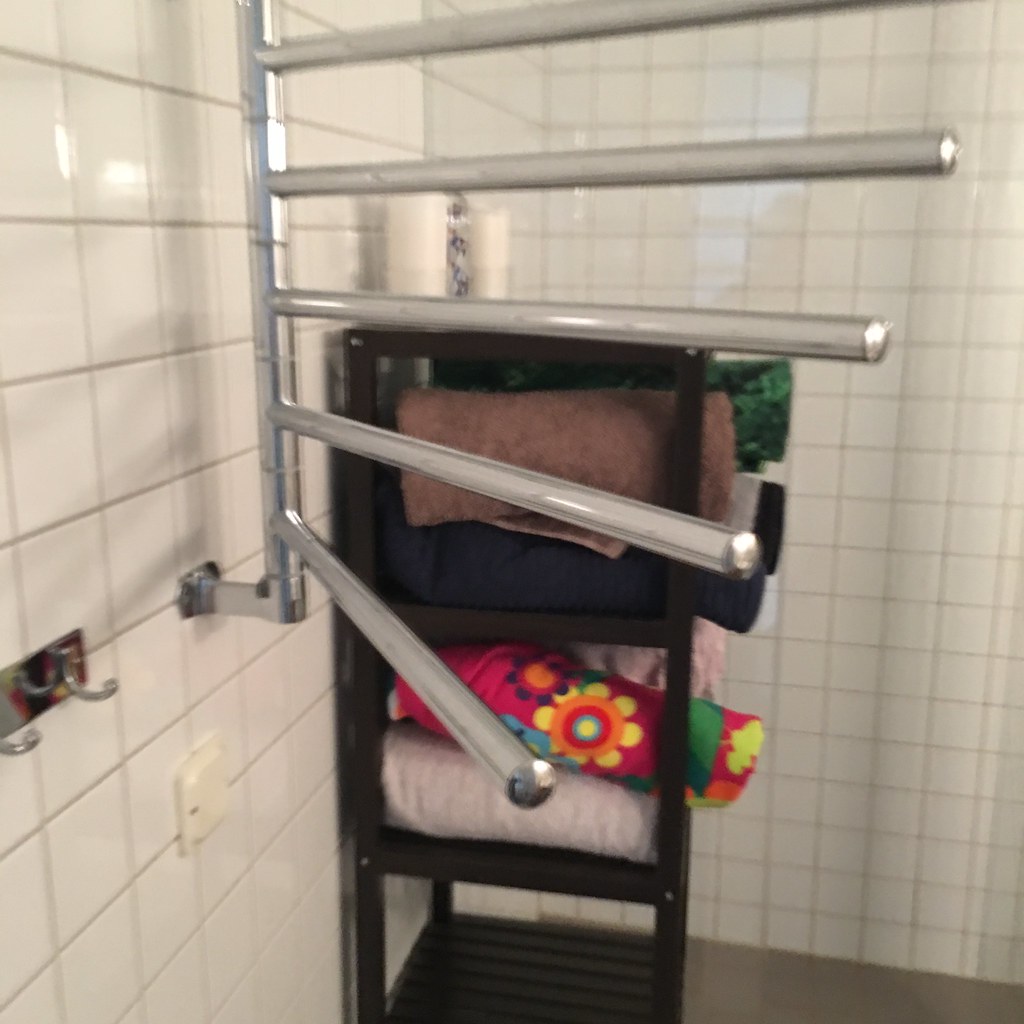This color photograph depicts a bathroom interior, featuring predominantly white tiled walls. The back wall, covered with smaller white tiles, contrasts slightly with the left side wall, which has larger white tiles. Positioned against the left wall, two metal hooks are mounted on a silver plaque, with nothing currently hanging from them. Slightly right of center, a unique vertical metal bar is affixed to the wall, from which five horizontal arms extend that can swivel for hanging towels; notably, the bottom arm is bent downward.

In the room's back corner, a black plastic shelving unit provides storage. This unit has four levels, with the bottom shelf empty and the remaining shelves neatly holding a variety of rolled towels. These towels come in an assortment of patterns and colors, including white, floral print, pink, brown, blue, a green leafy pattern, and black with gray. The cohesive elements of the image highlight the organized and utilitarian design of the bathroom, emphasizing the practical use of space and storage solutions.